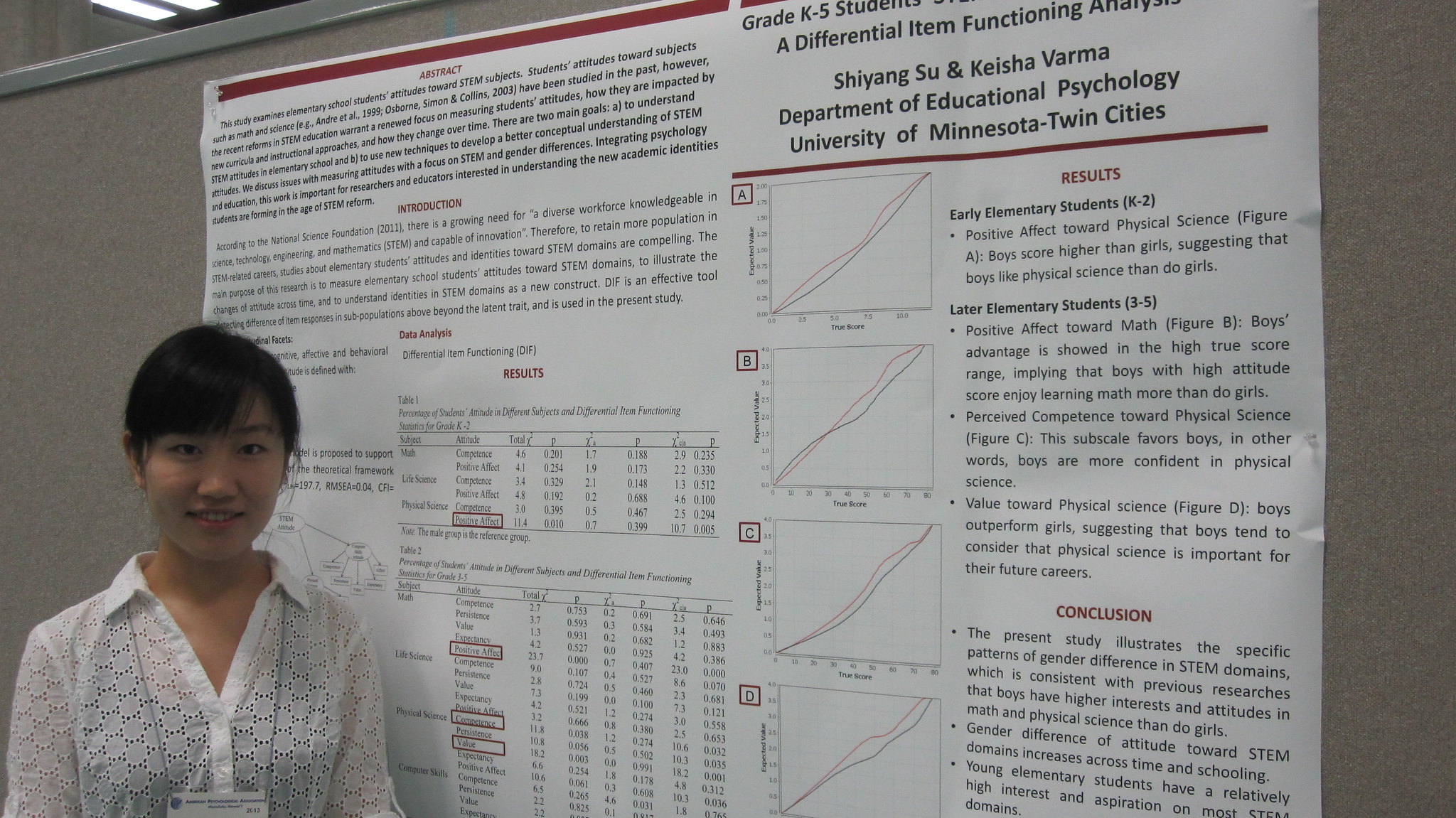In this horizontally aligned rectangular color photograph, a woman stands in the lower left corner in front of a tall gray cubicle wall. The upper left corner of the image reveals a sliver of background with a fluorescent ceiling light, suggesting an office or conference setting. The wall is adorned with a large white poster filled with small black text and red headings, summarizing the findings of a scientific study. Prominently at the top, centered on the left side, the poster begins with sections labeled "Abstract," "Introduction," "Data Analysis," followed by various charts and tables.

The poster details an educational study, titled "A Differential Item Functioning Analysis," and includes headings such as "Grade K-5 Students" at the top. The research is credited to Xiaoyang Su and Keisha Varma, affiliated with the Department of Educational Psychology at the University of Minnesota Twin Cities. The poster is divided with a thick red line separating the header from the detailed findings below, including line graphs with red and blue lines and sections labeled "Results" and "Conclusion," which contain bullet points and additional text.

The woman in the photo, likely one of the researchers, has short black hair with bangs and wears a patterned, slightly see-through white button-down collared blouse over a darker shirt. A white lanyard, presumably holding a name badge, hangs around her neck. She stands smiling, facing forward, adding a personal touch to the academic and analytical atmosphere of the scene.